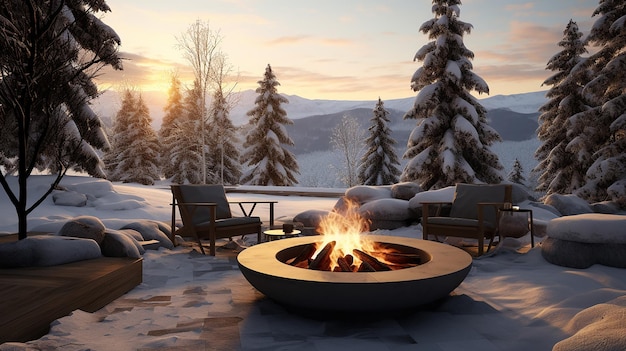The image is a horizontally oriented, rectangular scene depicting a picturesque winter landscape that might be either a realistic photograph or a digitally rendered image due to its smooth, animation-like quality. In the background, the sky is a blend of light blue and gray, with soft white clouds, and a bright, yellow sun is either rising or setting on the left, casting a warm glow. Snow-capped mountains stretch across the horizon, their peaks white and their bases darkening to black as they approach the foreground. 

Closer to the viewer are tall pine trees, their branches generously covered in snow, through which hints of green are visible. In the center foreground, a circular fire pit with a flat surface on top features neatly stacked logs radiating outward, supporting lively orange flames with light yellow cores. Surrounding the fire pit are two slightly oversized outdoor patio chairs with gray cushions and brown metal frames, positioned invitingly towards the fire. The ground around the fire pit is adorned with a light dusting of snow and scattered with large gray rocks. No people are present in this serene winter scene, which exudes a peaceful, natural beauty.